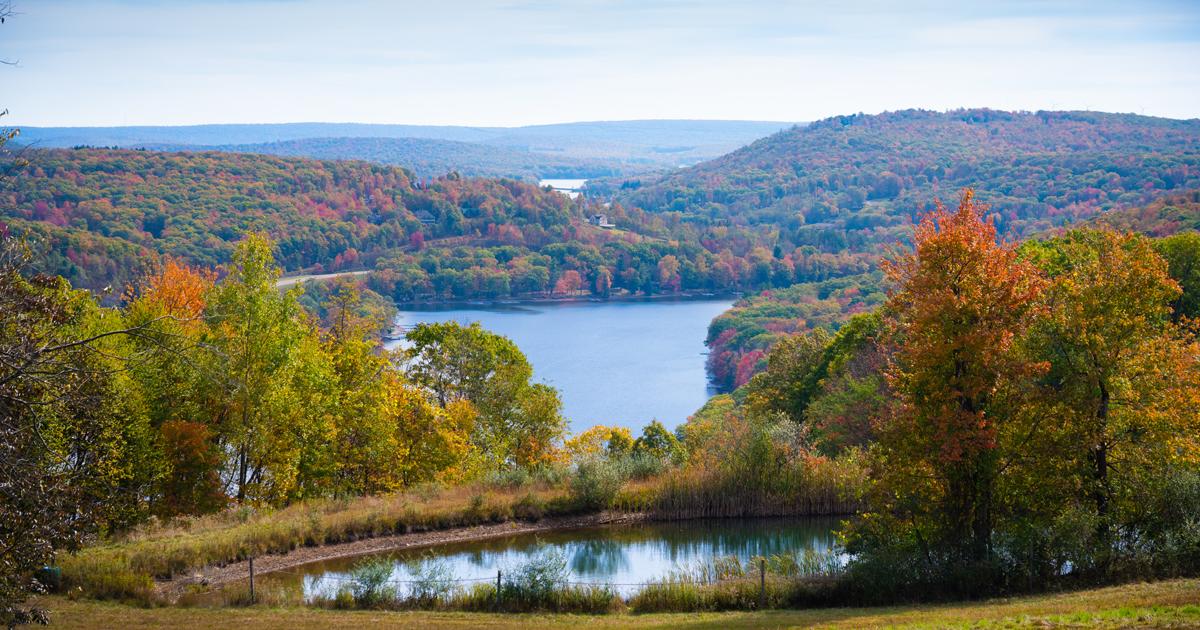This vibrant outdoor photograph captures a serene autumn landscape as viewed from atop a hill. In the foreground, a green hill slopes down to an oval-shaped, reflective pond encircled by a chain-link fence. This smaller body of water is nestled amidst deciduous trees beginning to change color, displaying a beautiful palette of green, orange, and gold. Further back, a larger, shimmering blue lake is surrounded by rolling, tree-covered hills, imbuing the scene with a tranquil, natural beauty. The sky above is bright and mostly clear, casting a gentle, hazy light over the entire landscape. In the background, near the base of the distant mountains, stand two man-made structures: a white building and a small house or barn, providing a subtle, human touch to this picturesque vista.